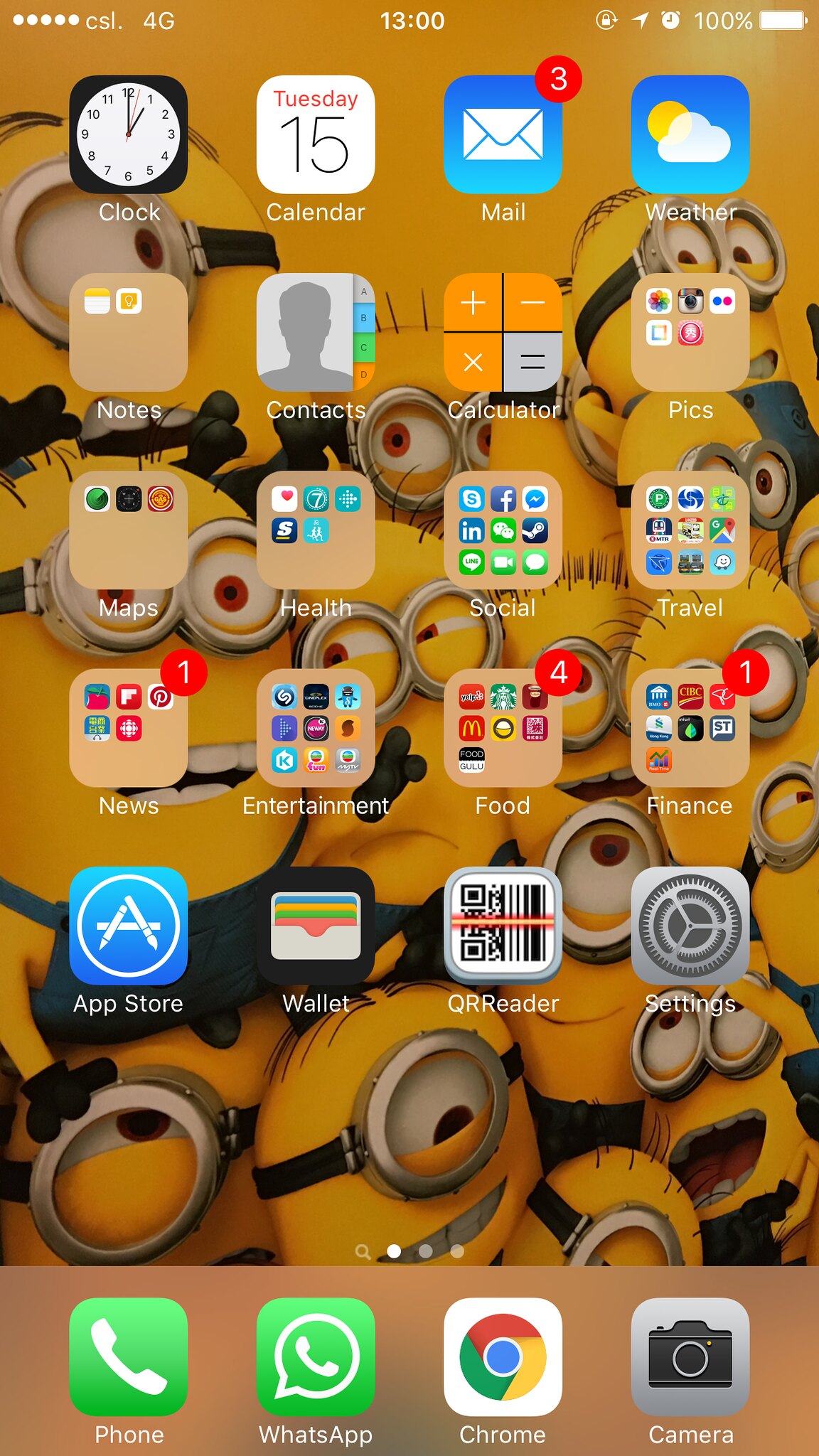This image showcases the home screen of a technological device, likely a smartphone. Here's a detailed breakdown of what's displayed:

1. **Top Bar:**
    - Five white circles.
    - "CSL dot" indicating network, alongside "4G."
    - Central white digital clock displaying "13:00".
    - A lock icon with a circular arrow around it.
    - Right diagonal arrow, clock symbol, indicating 100% battery power with a fully filled battery icon.

2. **First Row of Apps:**
    - **Clock**
    - **Calendar** displaying "Tuesday the 15th".
    - **Mail** with a notification badge showing three unread emails.
    - **Weather** featuring an icon of a cloud and sunshine.

3. **Second Row of Apps:**
    - **Notes**
    - **Contacts**
    - **Calculator**
    - **Pictures**

4. **Third Row of Apps:**
    - **Map**
    - **Health**
    - **Social** (inside which, apps like Skype, Facebook, WhatsApp, and Video are visible)
    - **Travel**

5. **Fourth Row of Apps:**
    - **News** with a notification badge showing one unread message.
    - **Entertainment**
    - **Food** with a notification badge showing four unread messages.
    - **Finance** with a notification badge showing one unread message.

6. **Fifth Row of Apps:**
    - **App Store**
    - **Wallet**
    - **QR Reader**
    - **Settings**

7. **Dock at the Bottom:**
    - **Phone**
    - **WhatsApp**
    - **Chrome**
    - **Camera**

Each app category on the screen is neatly organized with some having notification badges indicating pending messages or actions. The overall display is clear, showcasing essential apps and tools commonly used on a daily basis.